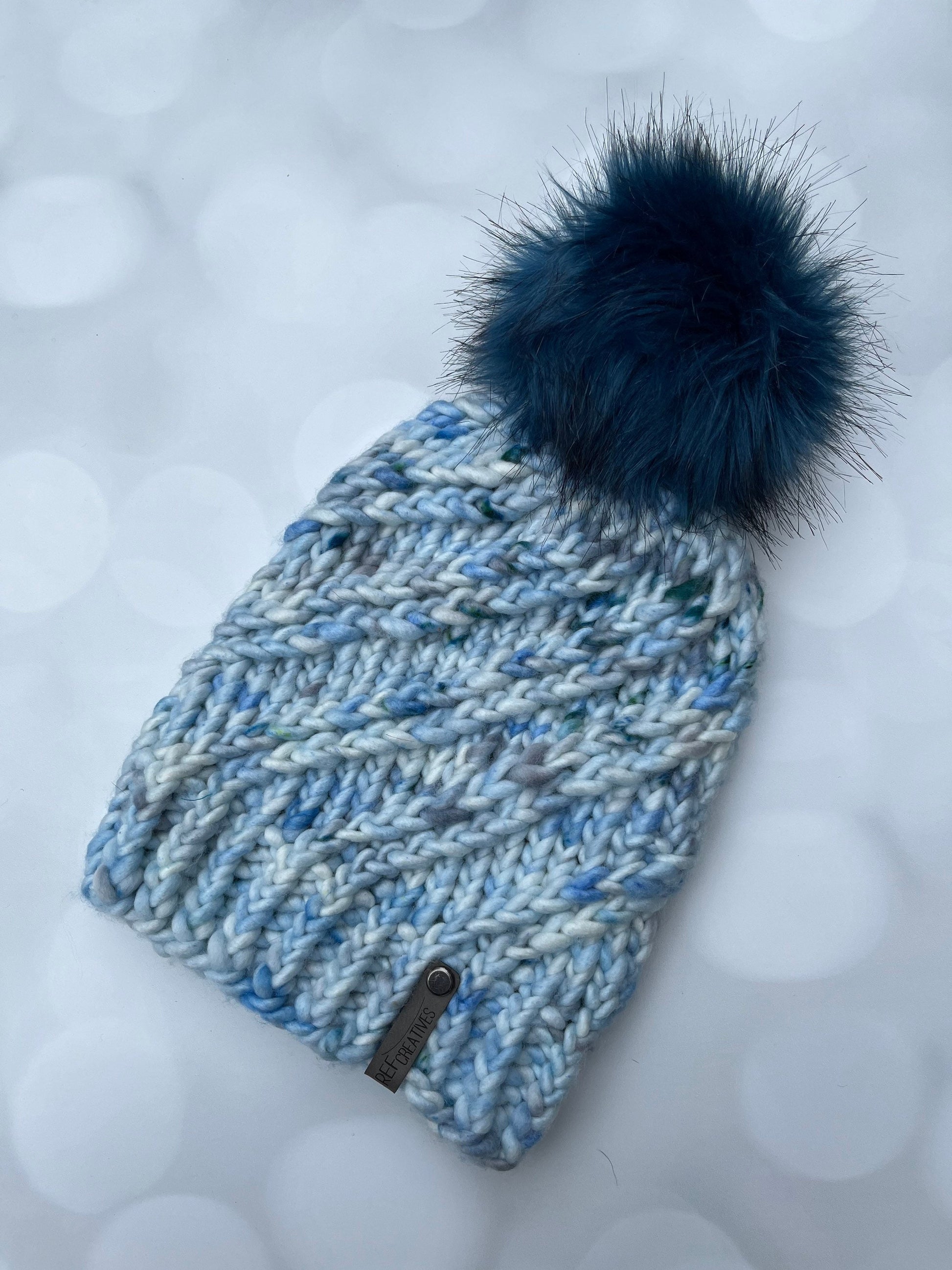The image is a vertically-oriented rectangular photo featuring a detailed view of a knitted winter beanie. The background is predominantly light gray with faint light gray circular areas reminiscent of flat bubbles, with a slightly darker shade in the bottom right-hand corner. Central to the image is a beanie, positioned at a slight angle, leaning towards the right roughly at the one o'clock position. 

This beanie showcases a navy blue, fuzzy pom-pom on the top, contrasting with its predominantly light blue, white, and slightly darker blue knitted fabric. The intricate knit pattern weaves diagonally from the bottom left to the top right. Additionally, there is a small, black tag located on the bottom right side of the beanie, possibly inscribed with the word "creatives" and featuring a button. The overall design of the beanie implies a snug fit, with the pom-pom being notably larger.